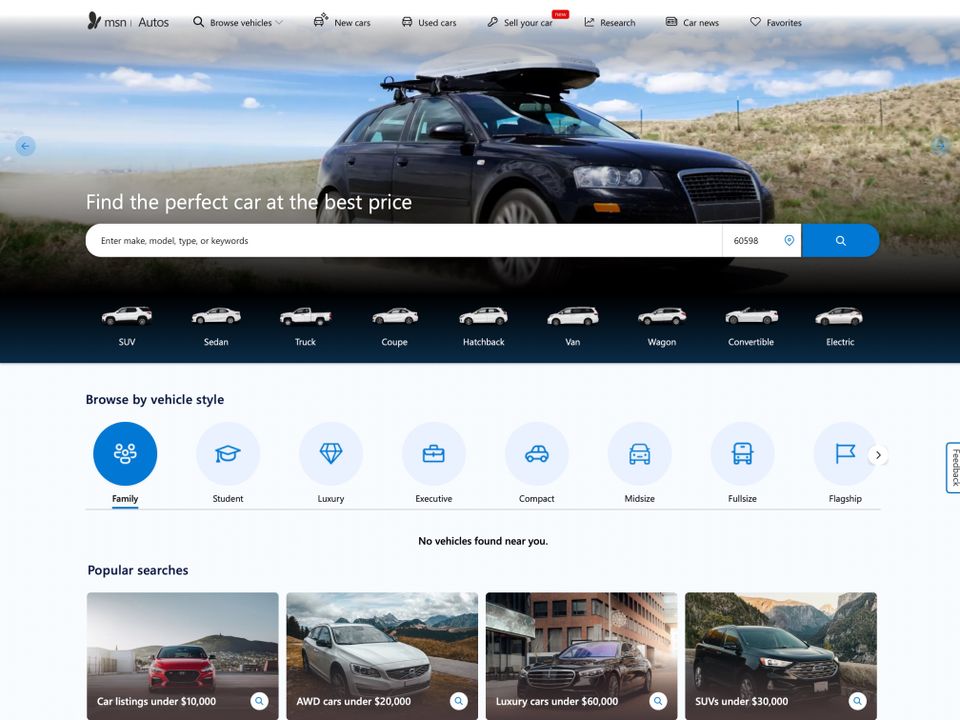The image showcases the homepage of the MSN Autos website. At the very top of the screen, the MSN logo is prominent alongside the word “Autos.” Below this, there is a comprehensive search facility for browsing vehicles, accompanied by a series of menu options which include New Cars, Used Cars, Sell Your Car, Car Research, Car News, and a Favourites section where users can save specific vehicles of interest.

Central to the layout is a large, striking image of a car navigating rugged terrain. This is paired with a prominent search dialogue box beneath it, encouraging users to “Find the perfect car at the best price.” Below this prompt, there is a variety of car shapes and models to choose from, such as SUV, Sedan, Truck, Coupe, Hatchback, Van, Wagon, Convertible, and Electric, allowing users to filter their search by vehicle type. Additionally, there is an option to browse by vehicle style, catering to needs such as Family, Luxury, Executive, and Compact cars.

Towards the bottom of the screen, there are convenient quick links categorized by price ranges, featuring options like Cars Under $10,000, Under $20,000, Under $30,000, and Under $60,000. These sections enable users to easily access popular and budget-friendly vehicle listings.